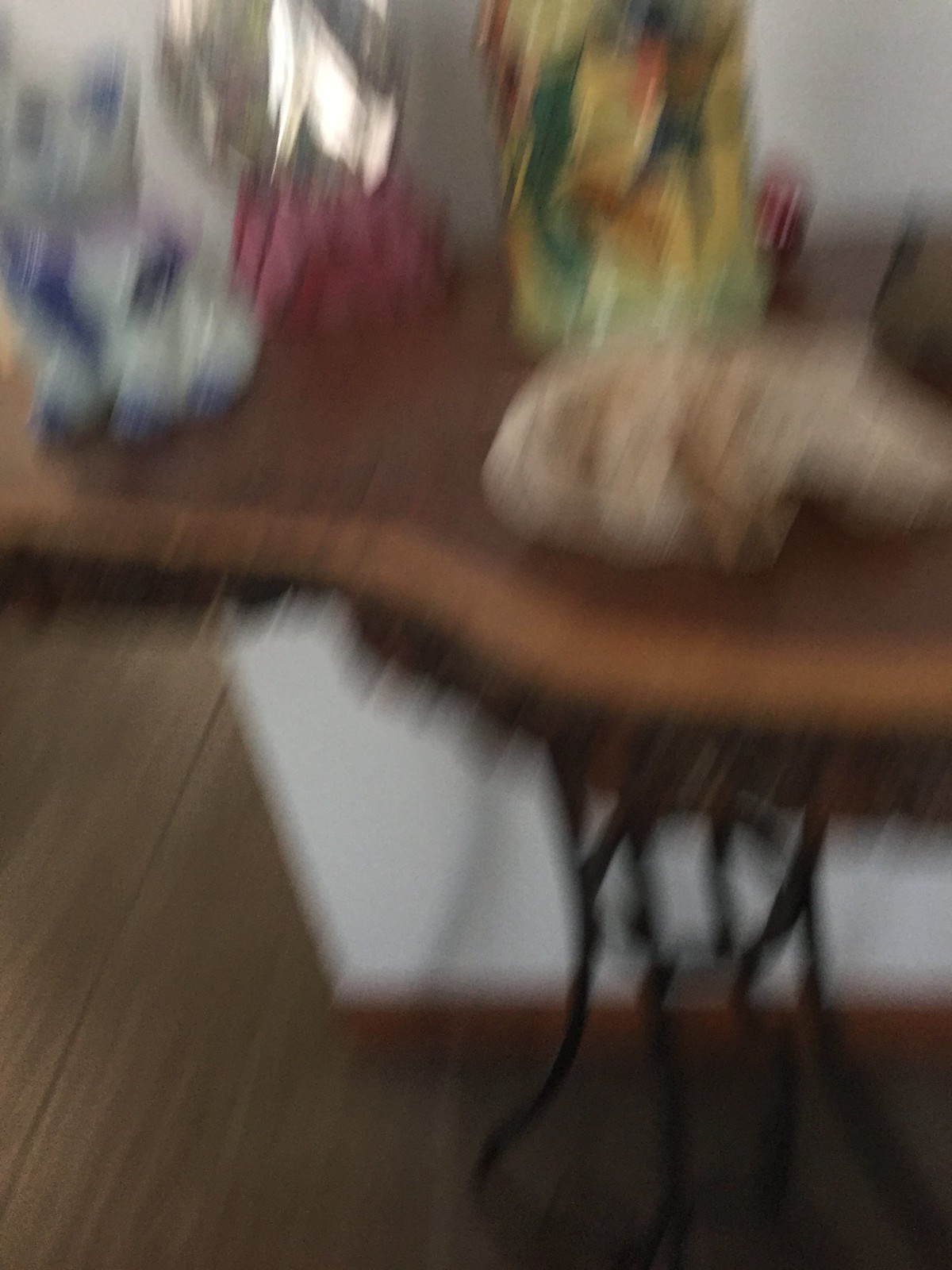This image is an extremely blurry, low-resolution photograph, making the details difficult to discern. The main subject appears to be a wooden table with a medium-colored wood top and black, possibly wrought iron or cast iron legs. The table is situated on a dark grayish wooden floor. There is a white, abstract-shaped object on the floor, perhaps a rug or a similar item.

On top of the table, several indistinguishable objects are visible. Among them, there is a beige object lying towards the front. To its left, there might be a small figurine resembling a puppy, white with bluish-purple details like feet and eyes. Adjacent to it, another taller object appears to have a pink bottom and silver top. Further towards the right side, a larger object is mainly yellow with green and orange accents, possibly resembling a gift bag or floral arrangement. Behind this, a smaller red item, potentially a candle holder, is partially visible. Despite the severe blurriness, these descriptions piece together a scene of a wooden table cluttered with various colorful objects.